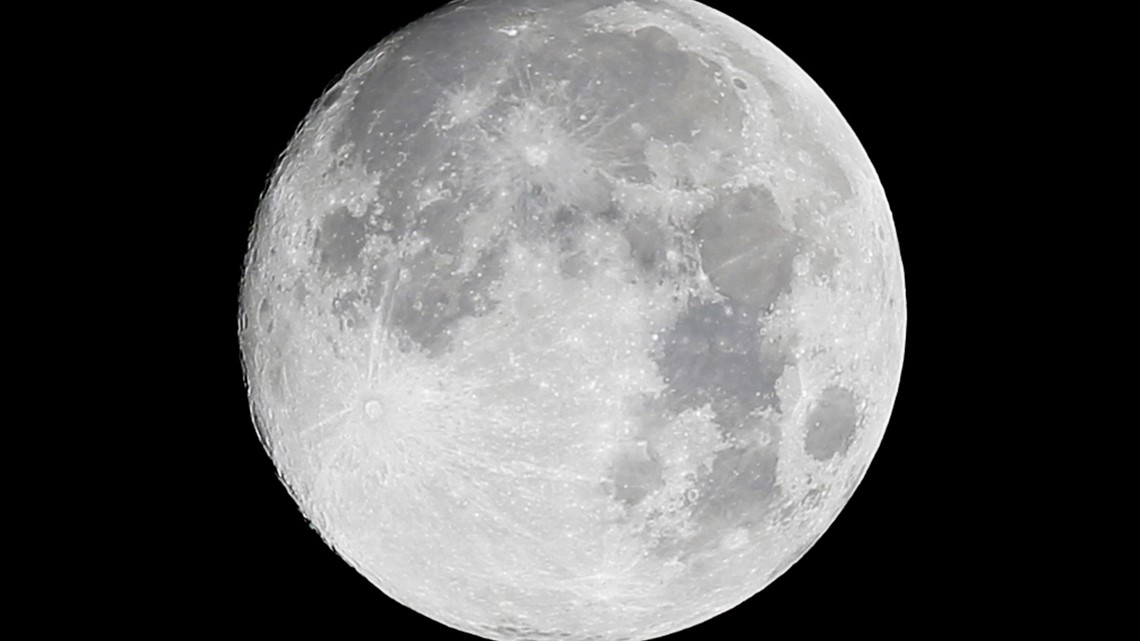This photograph depicts a striking full moon centered against an entirely pitch-black sky, devoid of stars. Due to the landscape orientation of the image, the very top and bottom edges of the moon are slightly cropped. The moon's surface is detailed with numerous craters, featuring varying shades of light gray and darker gray areas which highlight its rugged terrain. Prominent are the cratered regions that display white lines extending across, particularly noticeable on the left side. Larger, deeply colored craters are visible in the upper-middle and right sections, contrasting with the smoother parts of the moon. Scattered white glowing dots add to the surface's intricate texture. The overall composition emphasizes the moon's detailed surface while maintaining a stark contrast with the deep black surrounding space.